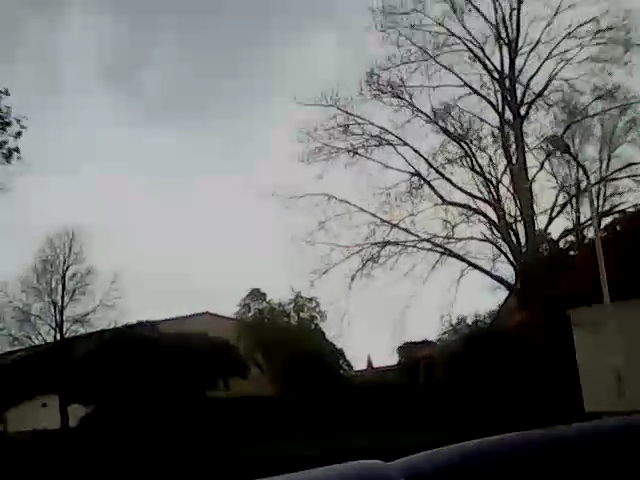This image captures a neighborhood scene under an overcast sky. In the right portion of the frame, there's a bare tree, devoid of any leaves, standing starkly against the muted backdrop. The center of the photo is occupied by several lush, green trees that are brimming with foliage, providing a striking contrast to the barren branches nearby. The image quality is notably low, characterized by visible pixelation, especially in the gradient sky above, which shifts from a light gray to a muted blue and then to a nearly white hue closer to the horizon. In the background, on the left side, a large white house with a pointed roof is partially obscured by the greenery. Additionally, a light pole stands on the right side of the image, emerging just beyond the leafless tree.